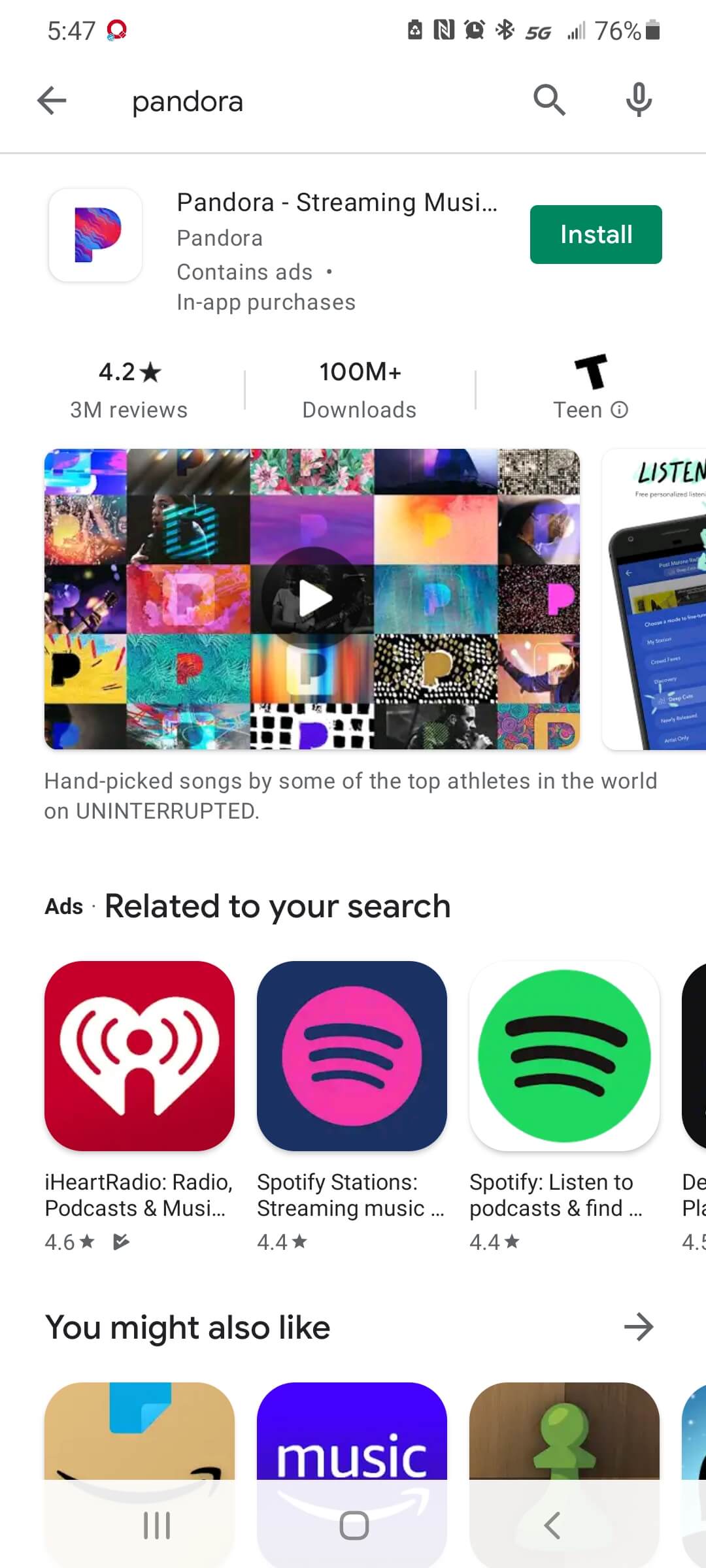A detailed screenshot description of a phone displaying the Google App Store page for the Pandora app:

The image is a screenshot taken from a smartphone at 5:47, showing the Google App Store interface for the Pandora music streaming application. Various icons and notifications populate the status bar: on the upper left, a program notification icon is visible. On the upper right side, notifications include an alarm icon, an active Bluetooth icon, a 5G connection status with three out of five bars, a battery at 75% with what seems to be a recycling notification beside it, and an additional unclear icon bearing "Z" which might be a reference to an unknown application or feature.

The primary focus of the screenshot is on the App Store page for Pandora. The search term "Pandora" is input into the search field, flanked by a back button on the left, a clear search button on the right, and a voice search button at the far right. The Pandora app entry showcases the Pandora logo positioned to the left, adjacent to a prominent green "Install" button with white text on the right side of the screen. Pandora is described as a music streaming app that includes ads and offers in-app purchases.

Further information provided includes a 4.2-star rating based on 3 million reviews, over 100 million downloads, and a rating of "Teen". Below this section, there is a visual collage of different Pandora app landing pages featuring a play button.

Scrolling down, the screenshot captures related app advertisements for iHeartRadio (radio, podcast, music), Spotify Station (streaming music), Spotify (listen to podcasts), and additional suggestions marked as "You'll also like" that include Amazon Music and an unrelated chess program. 

The bottom of the screen contains the standard navigation bar of the device, displaying the 'menu', 'home', and 'back' buttons.